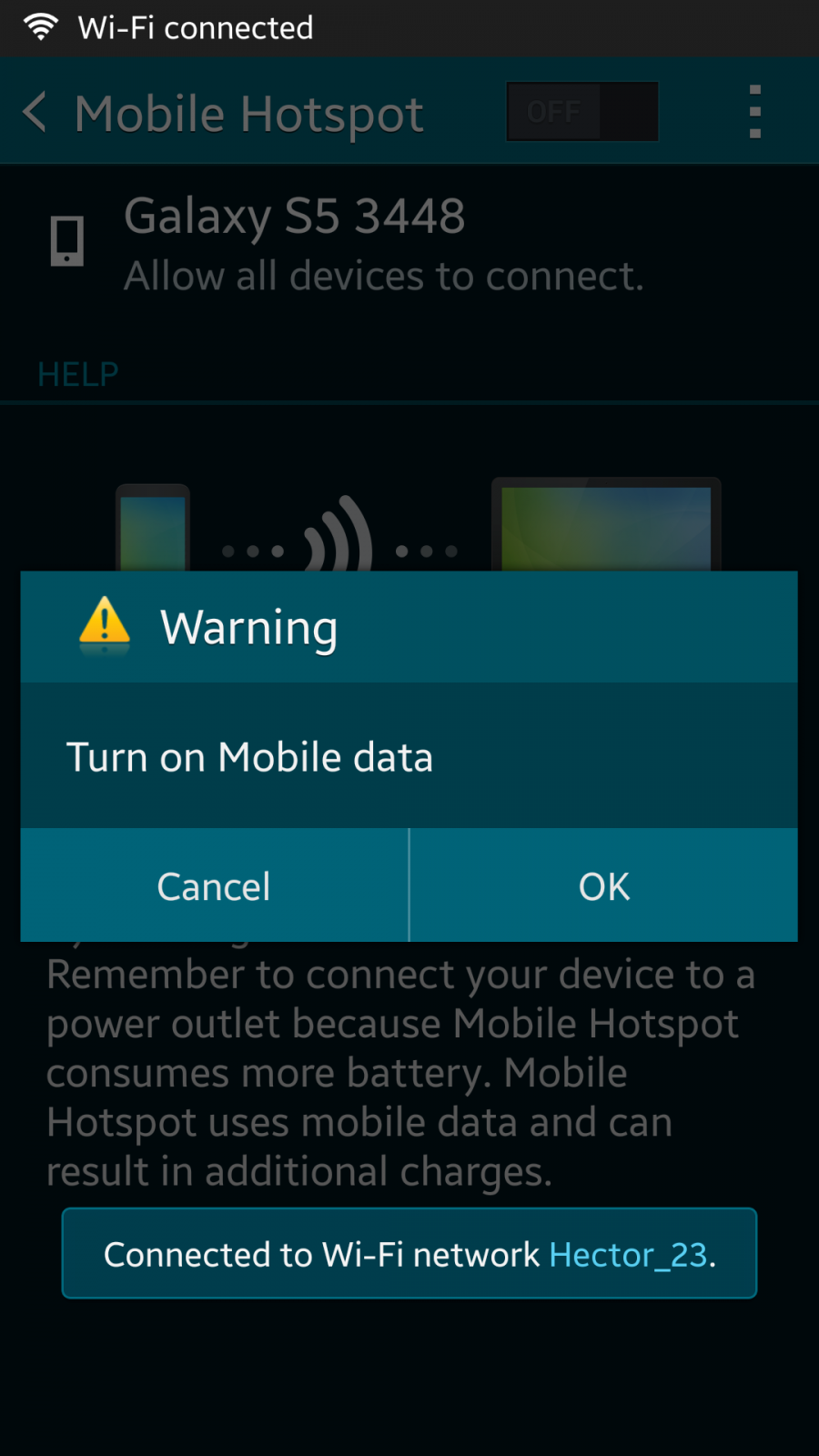The image features a predominantly black background overlaid with various graphical elements and text. At the top, there's a Wi-Fi symbol accompanied by the text "Wi-Fi connected." Below this, an arrow points left towards the label "Mobile Hotspot," situated next to a switch labeled "Off." Further down, a vertical ellipsis symbol is present.

Under these elements, a smartphone icon is displayed along with the text "Galaxy S5-3448." Following this, the text "Allow all devices to connect" appears, with "Help" written underneath. 

Towards the middle of the image, a dark blue pop-up button, featuring three different shades of blue, prominently displays a warning message. A yellow triangle with an exclamation mark icon and the text "Turn on Mobile Data" are prominently noted. Below this warning, there are two buttons: "Cancel" on the left and "OK" on the right. 

Further down, the text advises, "Remember to connect your device to a power outlet because Mobile Hotspot consumes more battery. Mobile Hotspot uses mobile data and can result in additional charges." 

At the bottom of the image, a blue box states, "Connected to Wi-Fi Network Hector_23."